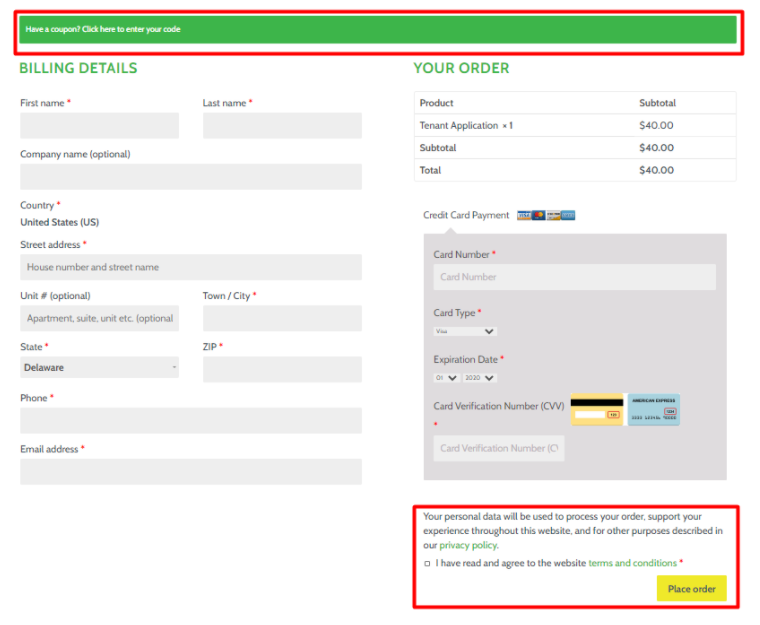This image depicts a detailed billing page from a website. At the top of the page, there is a prominent green bar that spans from left to right with the text "Have a coupon? Click here to enter your code," surrounded by an orange or red outline, prompting users to input their discount codes.

Beneath this bar, the section titled "Billing Details" is highlighted in green. The form below it features several gray input boxes for users to enter their personal information. This includes fields for first name, last name, company name (optional), country (defaulted to United States), street address, unit number, town/city, state, zip code, phone number, and email address.

To the right of this form, there is a section titled "Your Order." This section itemizes the user's selected products, showing a "Tenant Applications" product priced at $40. The subtotal and total amounts both reflect $40.

A darker gray box is provided for credit card information. Users are required to enter their credit card number, which is marked with a red asterisk indicating this field is mandatory. Additionally, users must select their card type from options including Visa, MasterCard, Discover, and American Express. Subsequent fields request the card’s expiration date and the card verification code (a 3-digit number found on the back of the card).

At the bottom of the page, a red box with white lettering informs users that their personal data will be used to process their order, support their experience on the website, and for other purposes as described in the website's privacy policy. The "privacy policy" text is clickable and highlighted in green. Users must also click to agree to the website’s terms and conditions.

Finally, there is a prominent yellow box labeled "Place Order," which users click to finalize their purchase.